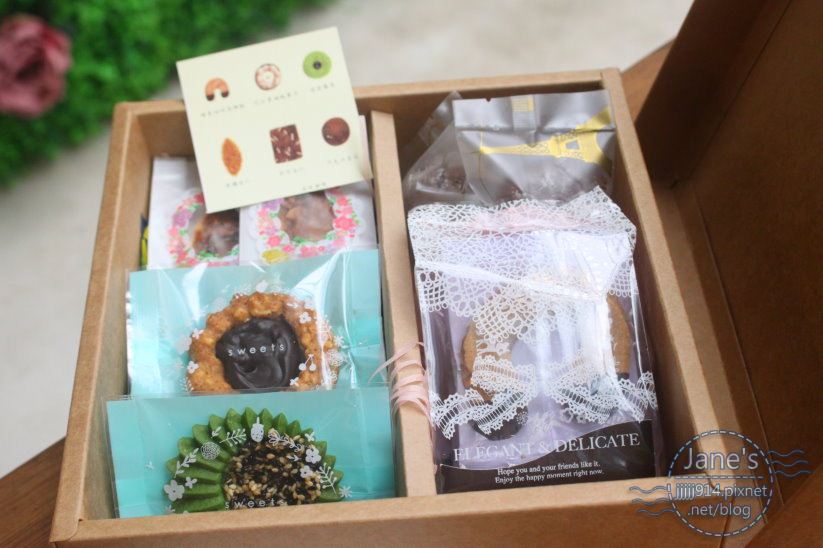This detailed photograph captures an elegant gift box, primarily made of wood, sitting on a wooden table. The box, which is rectangular, wider than it is tall, is open to reveal two compartments. The left side contains intricate, fancy chocolates and perhaps some cookies, all wrapped in plastic with blue and white packaging. One package distinctly reads "sweet," aligning with the box's overall theme of delicate desserts and treats. Various cookies of different shapes and colors are visible, including a green one, a light brown one with a black center, a brown leaf-shaped cookie, a rectangular one, and a simple brown circular cookie, accompanied by a small light brown card describing them, though the text is not fully legible.

The right-hand side of the box also contains more of these elaborate sweets, though the packaging here appears even more refined, marked by an inscription that reads "elegant, delicate." 

The image has a watermark in the lower right corner from Jane's, a company that perhaps specializes in such gourmet treats, with the URL jjjjj914.pixnet.net.blog. Additionally, imposed text in the lower right corner says "Jane's," suggesting the brand or store associated with these delicacies. A pink flower with green leaves is visible on the ground in the upper left corner, adding a touch of natural charm to the scene.